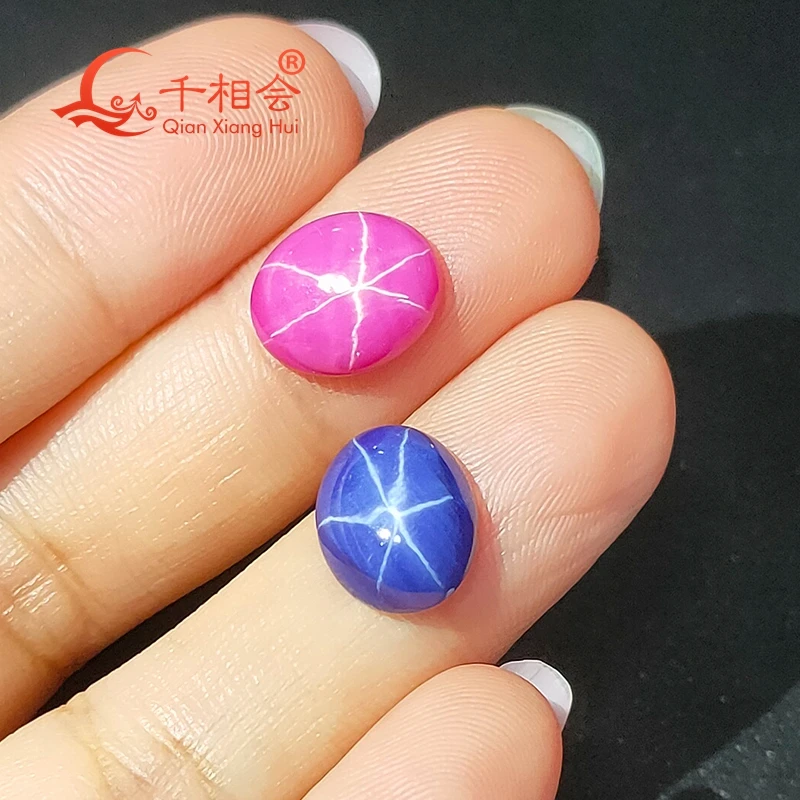A color photograph captures a close-up of fingers adorned with polished, semi-precious stones against a black backdrop. The hand, palm-up with long white fingernails, displays the index, middle, ring, and pinky fingers, though the thumb is not visible. The skin details and lines are clearly etched on the fingers. On the middle finger sits a fuchsia stone with white lines forming a star-like pattern, while the ring finger cradles a blue stone with similar white lines. Both stones, round and shiny, reflect light, creating a white center. Overlaying the index finger are red oriental characters, forming part of a logo. Additional red text appears on the upper left, contributing to the intricate visual details of the image.